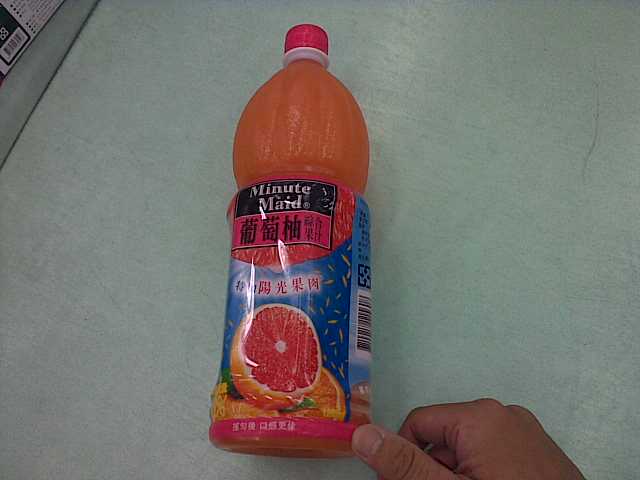In this grainy photograph, a pale gray countertop serves as the backdrop, partially covered by the thumb and knuckles of a hand extending from the lower right corner. The thumb touches a horizontally lying, unopened Minute Maid plastic bottle of juice sealed with a red cap. The label features the brand name "Minute Maid" prominently displayed against a black background, accompanied by colorful graphics, including a partially sliced grapefruit, hinting at the contents being grapefruit juice. Additionally, below the brand name, a phrase in an Asian script appears, suggesting a non-English product variant. The predominantly blue and pink label adds vibrancy to the otherwise muted and grainy scene.